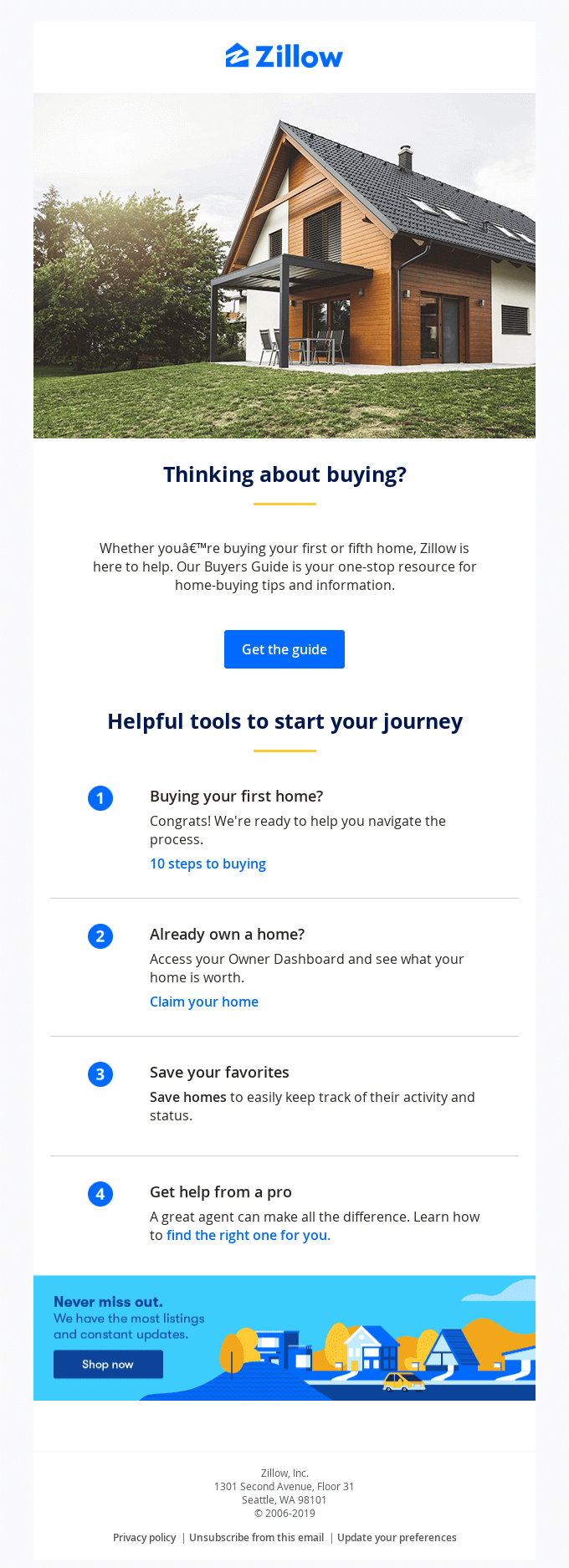This is a full-page screenshot from the Zillow website. At the top, a white banner prominently displays the centered word "Zillow." Below this banner, there is a large, vivid image showcasing the front exterior of a barn dominium-style house. Just beneath this image, the bold text "Thinking about buying?" immediately captures attention. Below this text is a small, double-spaced yellow line.

Further down, there is a brief descriptive text, followed by a centered blue box with the prompt "Get the quote" set against the backdrop of the house image. Moving lower, the page features another section title, "Helpful tools to start your journey," written in bold blue font.

Beneath this, a vertical list of four items is displayed, each numbered from 1 to 4 on the left side. Similar to the previous yellow line, these numbers are highlighted with a double-spaced yellow bar.